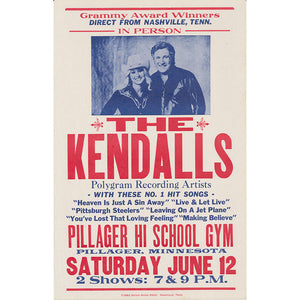This event flyer announces a live performance by Grammy Award winners The Kindles, direct from Nashville, Tennessee. The flyer, primarily set against a white background with red and blue lettering, highlights the duo's musical achievements as Polygram recording artists with a list of their number one hits including "Heaven is Just a Sin Away," "Live and Let Live," "Pittsburgh Steelers," "Leaving on a Jet Plane," "You've Lost That Loving Feeling," and "Making Believe." The main headings and crucial information are accentuated in red font. 

The flyer showcases a photograph of the band members: a smiling woman wearing a cowboy hat and a country shirt, and a man in a satin-style cowboy outfit with his arm affectionately draped around her. The event is scheduled to take place at the Pillager High School Gym in Pillager, Minnesota, on Saturday, June 12th, with two shows at 7 p.m. and 9 p.m. The visual layout suggests it is designed for easy posting on community boards or telephone poles, ensuring widespread visibility.